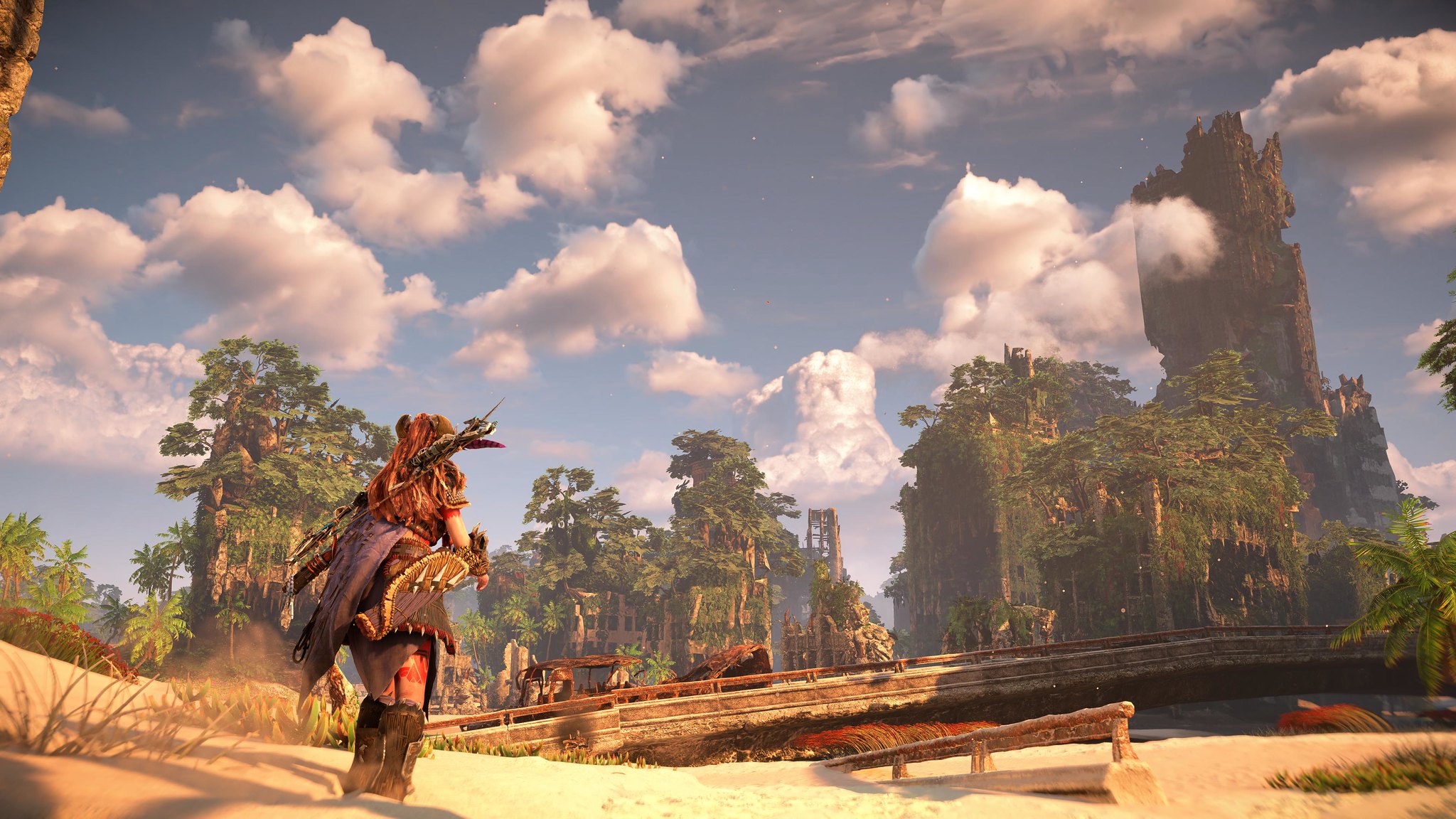In this screenshot from a highly detailed and realistic video game, a female character with long red hair is depicted standing on the left side of the image. She is armed with a bow and arrow slung across her back, gazing towards the backdrop of the scene. The background reveals a dystopian cityscape with tall, dilapidated tan buildings overrun by lush greenery, emphasizing their age and state of abandonment. The character is positioned on light tan sand, suggesting a desolate, post-apocalyptic environment. Directly in front of her is a decrepit, rust-colored bridge, partially disintegrated and adorned with tones of gray and tan. Upon the bridge sits an old, rusted car, further highlighting the scene’s theme of decay and neglect. The overall composition conveys a sense of adventure and survival in a world reclaimed by nature.